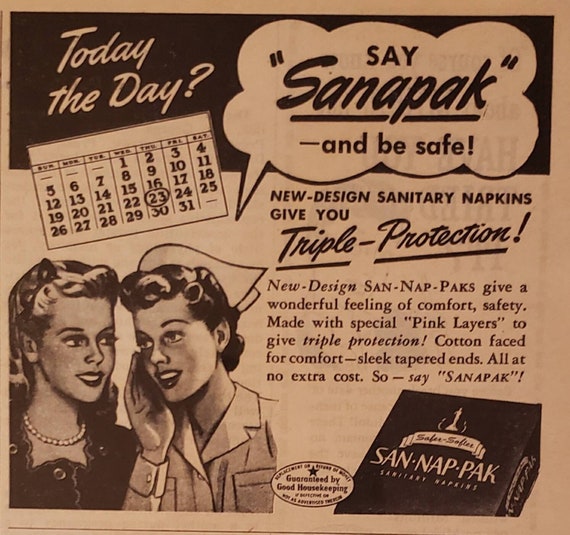This detailed vintage advertisement for Sanitary Napkins, now faded to a pink hue, features prominently in the image. It showcases the slogan, "Today's the day? Say Santa Pack and Be Safe." In the upper left corner, a calendar with the date "23" circled underscores the urgency of the message. Below this, two young women, one dressed as a nurse and the other presumably a consumer, lean in towards each other, smiling, highlighting the trust and camaraderie associated with the product. The lower section of the advertisement boasts, "New Design Sanitary Napkins give you triple protection," and includes an image of the SanNapNPak box in the lower right corner. The detailed description cites the product's benefits: triple protection through specially designed pink layers, cotton facing for comfort, and sleek, tapered ends, all offered at no additional cost.